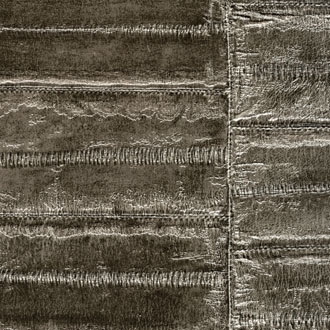The image depicts a nondescript, metallic-looking object with a predominantly brownish-gray color. It features a shiny, smeared surface divided into sections by various white, squiggly lines. Most of these lines are located on the far-right side of the image, with one predominant vertical line that runs three-quarters of the way toward the right edge. This line creates a clear division, with six smaller sections on the left and three on the right. The surface has a textured, wrinkled appearance, akin to melted and stamped metal but without any distinct figures or writing. The overall visual impression is one of a flat, gleaming material segmented by ridges and indentations, creating an abstract pattern with no clear identifiable entities, evoking a sense of ambiguity.